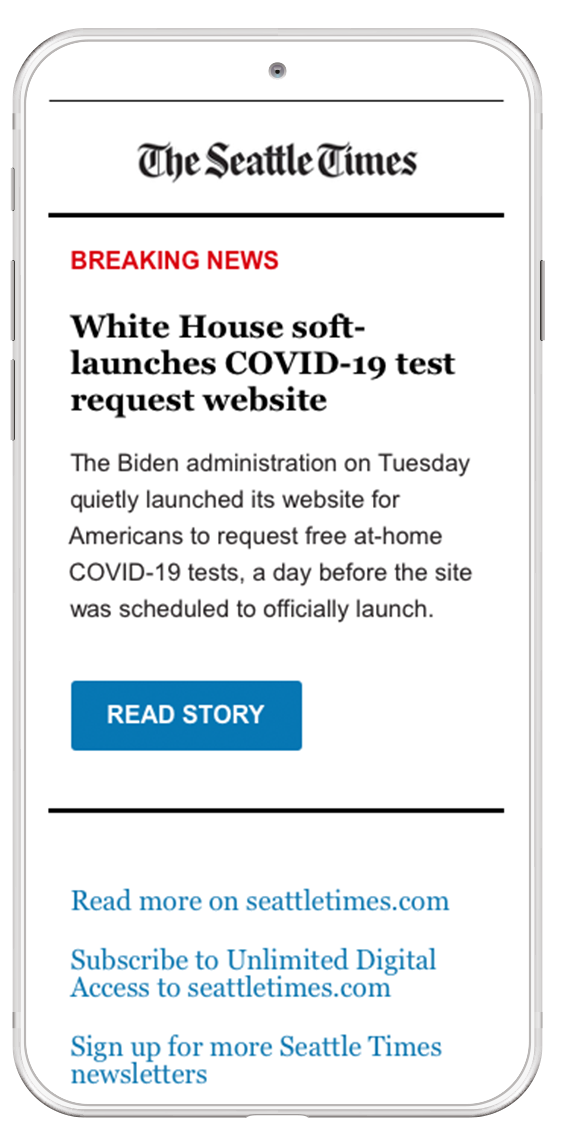A smartphone screen displays a Seattle Times article framed by white borders. At the top of the screen, there is a "Breaking News" banner in red text against a white background. The headline reads "White House Soft Launches COVID-19 Test Request Website." Below the headline, it states that the Biden administration quietly launched a website on Tuesday for Americans to request free at-home COVID-19 tests, one day prior to the official launch date. In the center of the screen, there's a blue rectangle with the prompt "Read Story." Further down, black text provides more details, followed by blue text offering options to "Read more on seattletimes.com," "Subscribe to unlimited digital access to seattletimes.com," and "Sign up for more Seattle Times newsletters." The smartphone features three buttons on the left side and one button on the right side, with a slit for the camera at the top edge, framing the article.